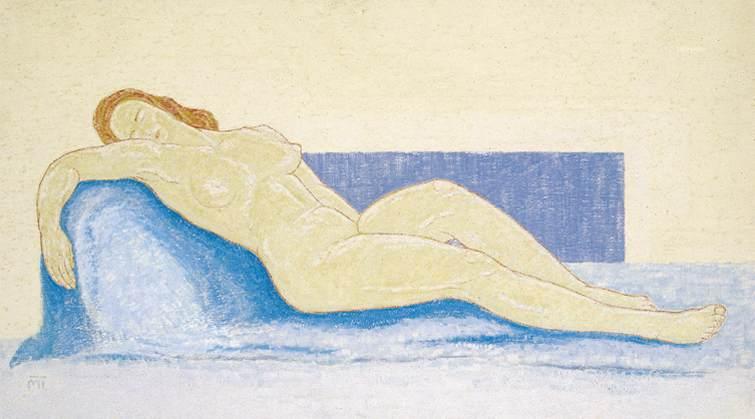The image is a detailed hand-drawn artwork on a beige canvas, employing what appears to be colored pencils or pastels. The focus is a nude, light-skinned Caucasian woman with long brown or auburn hair, who is lounging in a reclining position. She lies against a blue shape that could resemble a rock, a recliner, or a couch, transitioning from dark blue at the edges to lighter blue in the center. The woman's head is turned to the left with closed eyes, resting on her shoulder, and her legs extend to the right, with one leg slightly drawn up. Her left arm is draped over and down the side of the blue shape, while her other arm is obscured from view. The surrounding scene includes a blue blanket draped underneath her and over a white bed, with a light, textured brown background. A purple square appears behind the bed, adding depth and contrast to the scene. The overall depiction suggests a serene and relaxed state, emphasizing the gentle contours and subtle shading of the medium used.